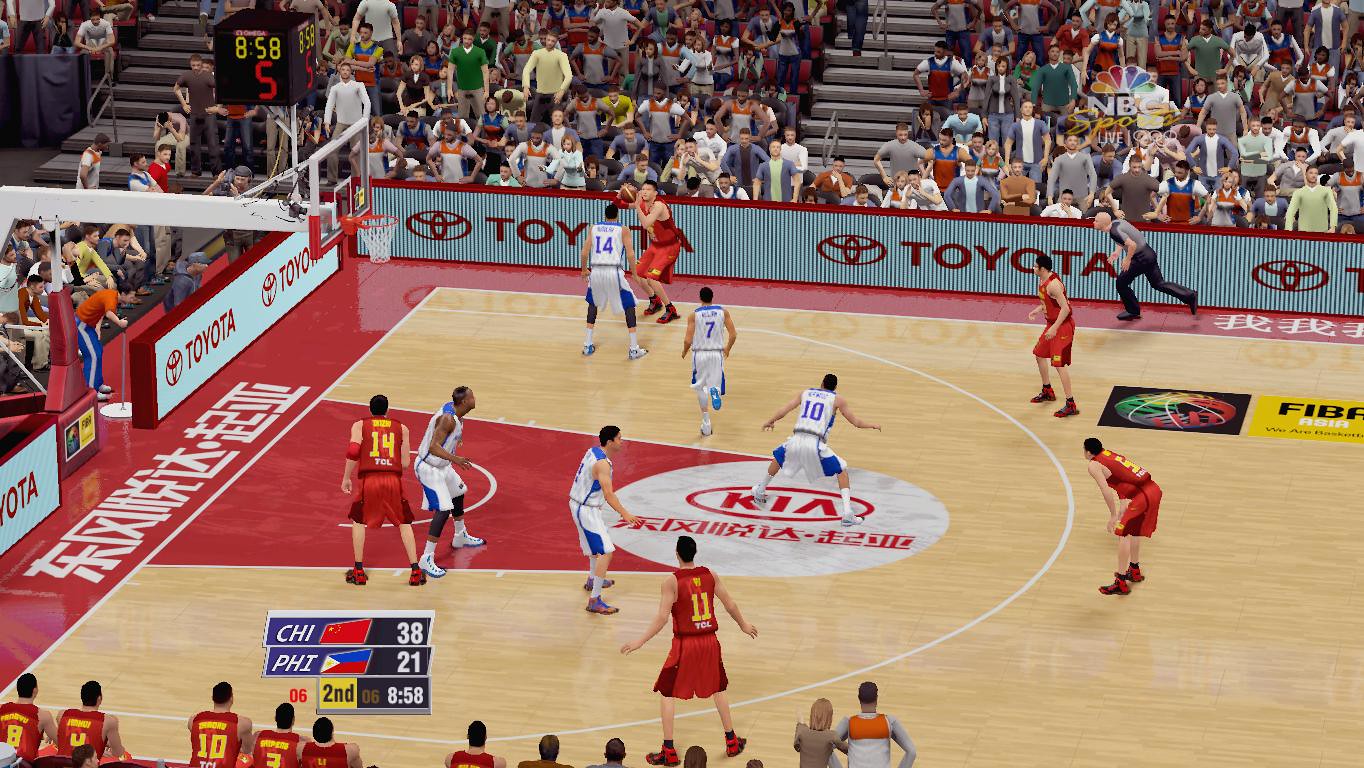This image is a detailed still from a basketball-themed video game set inside a bustling stadium. The scene showcases two competing teams, one in red uniforms with yellow numbers and trim, and the other in white uniforms with blue accents. The court has a traditional design with a tan coloring and a prominent red paint area, featuring a white circular zone near the free-throw line with the word "Kia" in red, accompanied by Chinese characters. 

Overhead, a shot clock displays "858" in yellow font, indicating the time left in the second quarter, with a large red '5' for the shot clock. The left side of the court is abuzz with an animated audience, some standing and others seated. Advertisements, mainly for Toyota, line the rectangular edges of the court, characterized by white backgrounds, red borders, and red text.

On the court, the main action features a player from the red team poised at the three-point line, preparing to make a shot, while number 14 from the white team attempts to block him. Additional players, including numbers 7 and 10 from the white team, are strategically positioned to defend against the red team. At the bottom left of the image, a score graphic indicates CHI leads with 38 points over PHI, which has 21 points, suggesting the teams could be China and the Philippines.